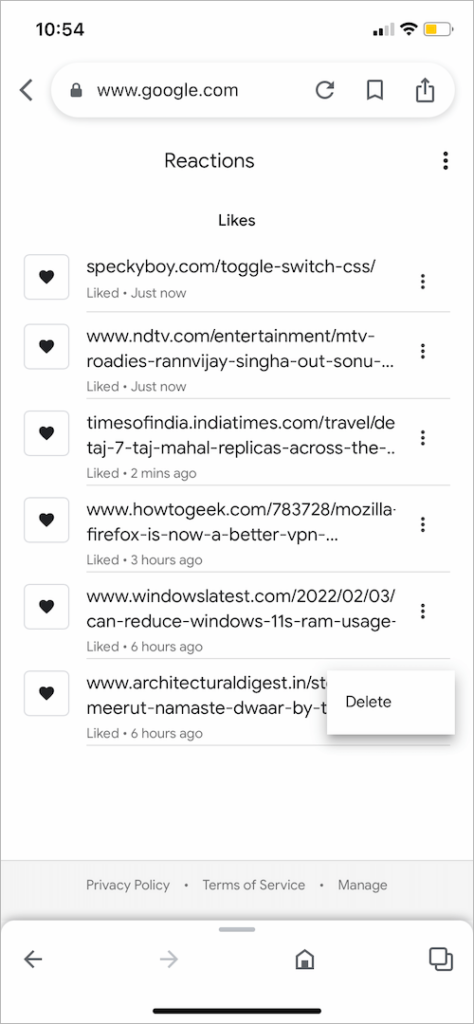Screenshot of a Mobile Device Displaying Google Search Results:

The screenshot, taken at 10:54 AM, shows a mobile device interface. The carrier signal is indicated by two bars and Wi-Fi is enabled, with the battery level at approximately 35%.

At the top of the screen, the Google search bar displays "google.com," alongside icons for refresh, tabs, and sharing options. A padlock symbol indicates the webpage is secure. 

Centrally, the screen features a section titled “Reactions,” showcasing several liked items. The background is white with black text. The first item is a link to "Speckyboy.com/toggle-switch-CSS," marked "liked just now" with a heart icon. Subsequent items include:
- www.ndtv.com/entertainment/mtv-roadies-ranvijay-singa-out
- Times of India
- How to Greek
- Architectural Digest

All are accompanied by heart icons, denoting they have been liked.